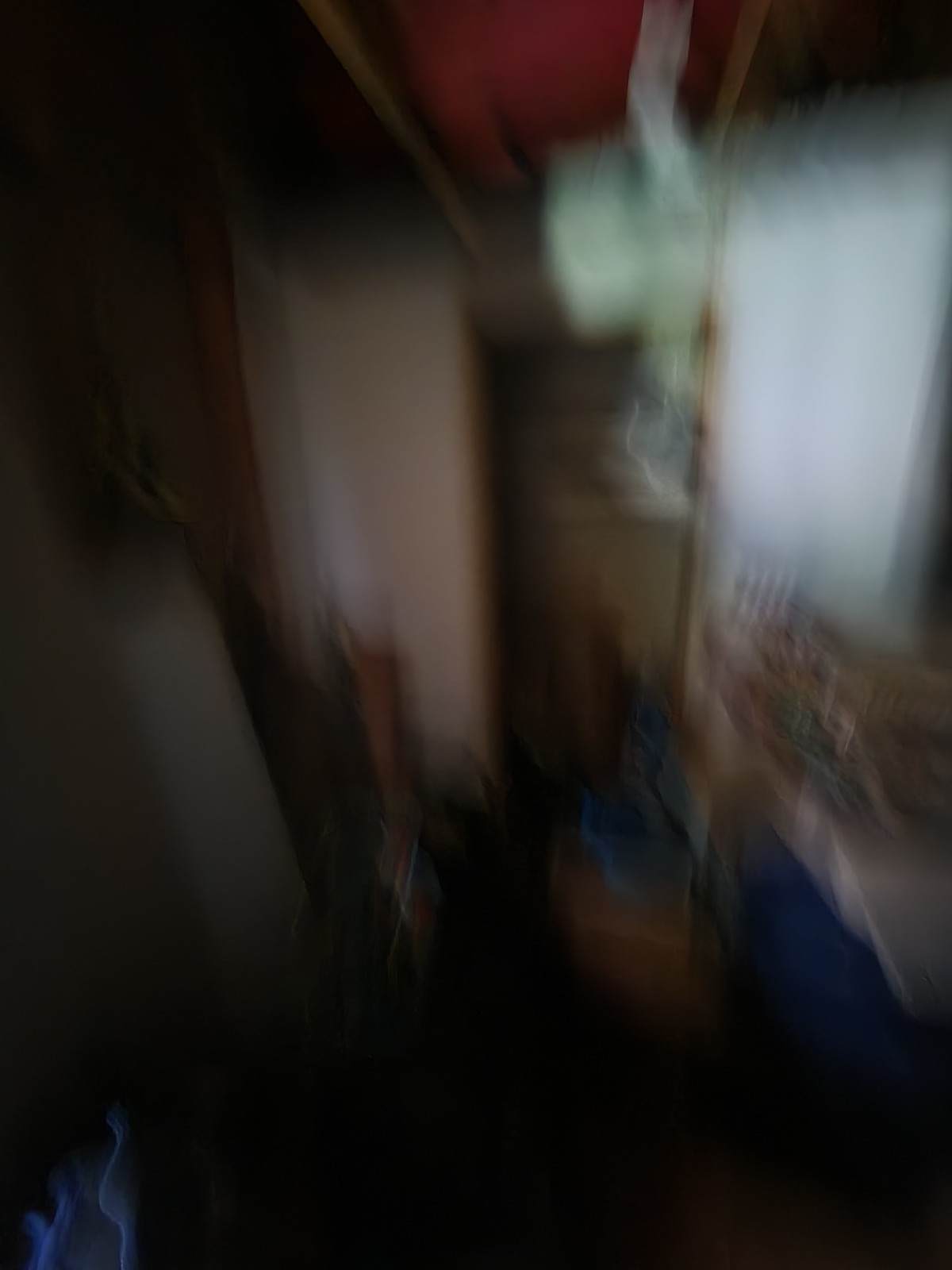This image features a dimly lit and significantly blurry view of an interior space, likely a house. The scene is dominated by dark tones with a few discernible elements. A white wall encloses the main area, while the ceiling has a red object attached, contrasting against its dark brown hue. A white curtain, faintly illuminated by sunlight, hangs in the background. In the bottom left corner, there is a blue light source resembling a flame, though it is not an actual flame. The bottom right corner reveals what seems to be a bed, covered with a blue sheet and possibly bearing an object on top. Centered in the room is a box, with an open door nearby, likely leading to a closet rather than stairs.